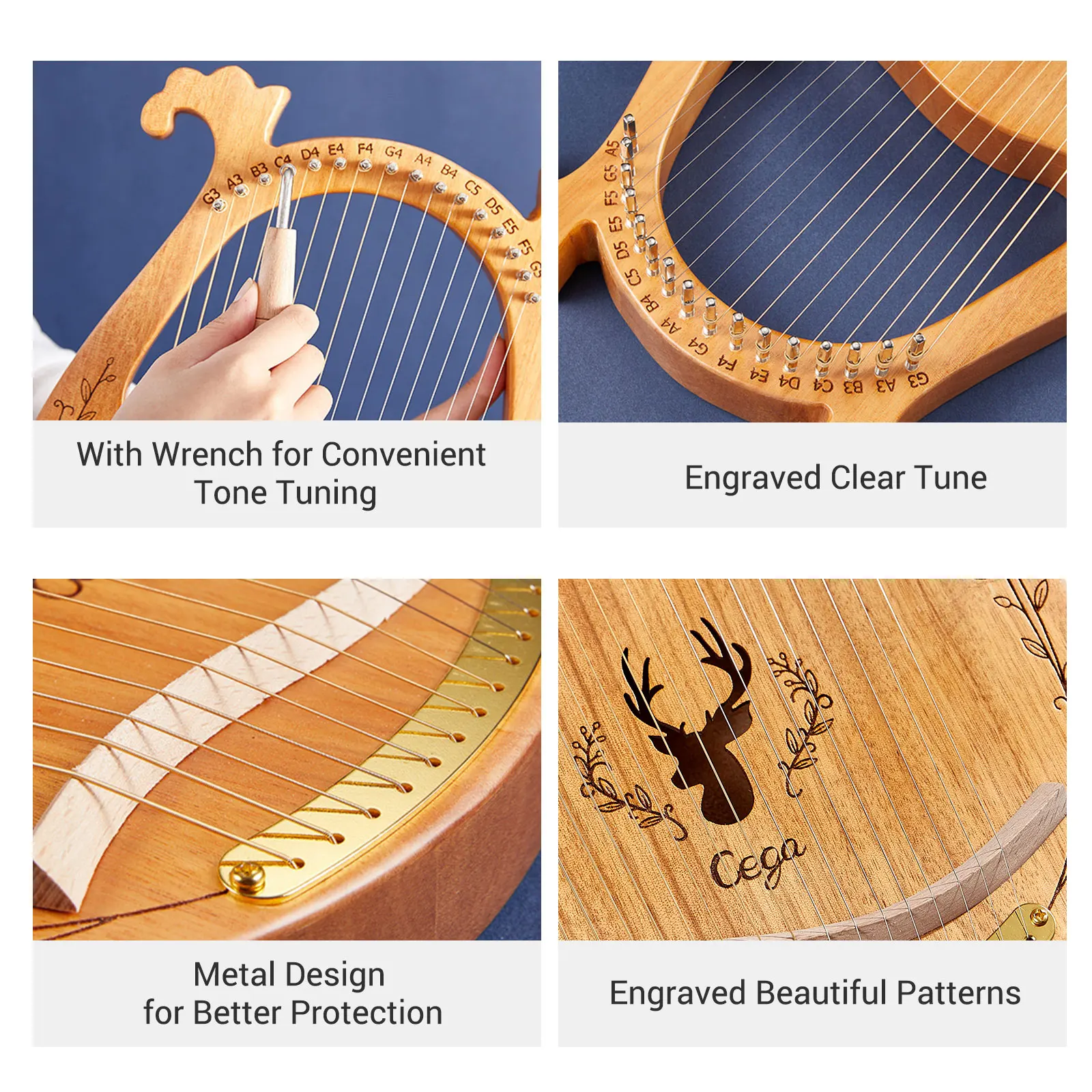The image comprises four distinct quadrants, each illustrating different aspects of a wooden hand-held harp. The quadrants are arranged in a grid format with a white cross separating them. In the top left quadrant, a person's hand is shown using a wrench to tune the strings, with the text "With wrench for convenient tone tuning" underneath. The harp has notes labeled on the strings, ranging from G3 to G5. The top right quadrant features the harp lying on its side, showcasing the labeled strings and the text "Engraved clear tune." 

In the bottom left quadrant, a close-up reveals the metal plate at the base of the harp where the strings are secured, accompanied by the text "Metal design for better protection.” The metal plate appears to be of higher quality, possibly gold or brass, ensuring durability and protection for the instrument. The bottom right quadrant displays an ornate engraving of a deer head with large antlers and vines around it, along with the text "Engraved beautiful patterns." Below the engraving, a name written in cursive, possibly "CEGA" or "SEGA," adds a personalized touch to the instrument. The harp itself is crafted from light-colored wood, further emphasizing its elegant and detailed design.